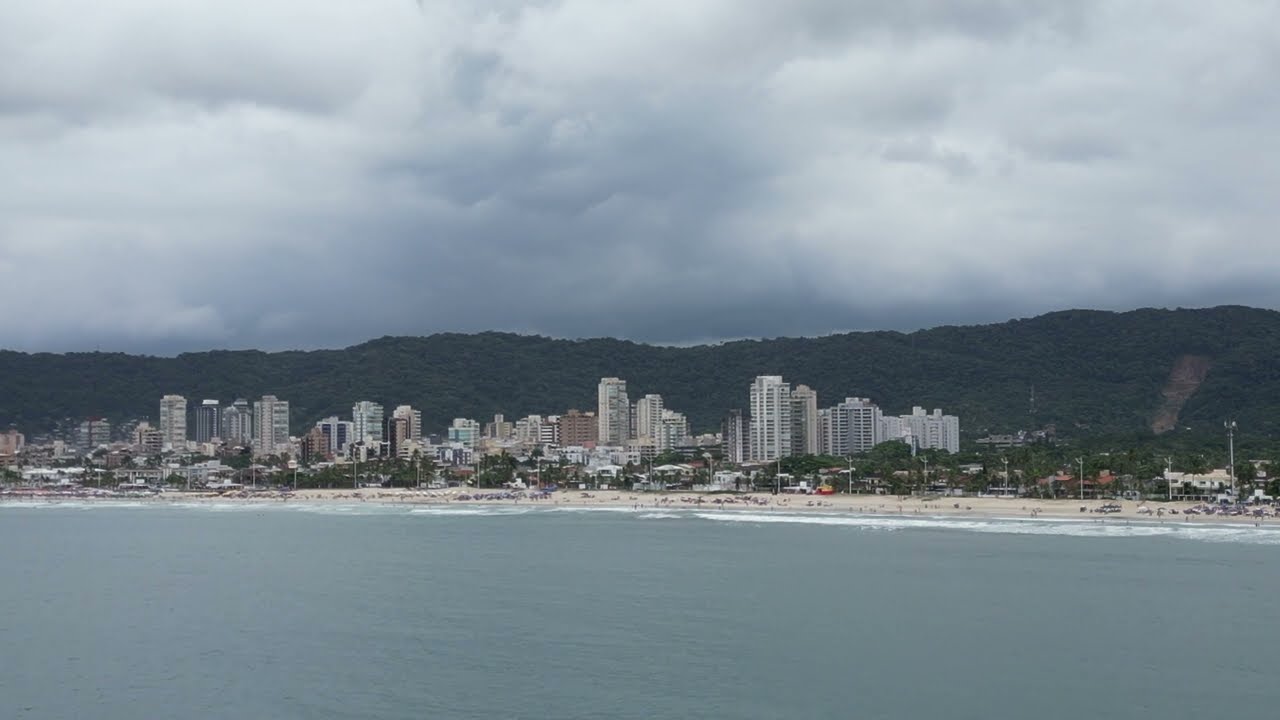This panoramic, postcard-style photograph captures a bustling beachside cityscape. The image, wide in length and short in height, is taken from just offshore, looking towards the coastline. A white sandy beach stretches across the foreground, dotted with numerous beachgoers enjoying the cloudy, potentially rain-threatening day. Gentle waves crest with whitecaps as they approach the shore. 

Dominating the midsection are an array of beachfront buildings, ranging from modest five-story structures to towering skyscrapers, likely encompassing hotels, apartments, and condos. These buildings display a palette of white, brown, and gray, standing in stark contrast to the lush, tree-covered hills that form the backdrop. The verdant hills span the width of the image and add a sense of depth and natural beauty to the urban landscape. The overall scene is captured under a blanket of gray clouds, contributing to the photograph's muted yet captivating atmosphere.